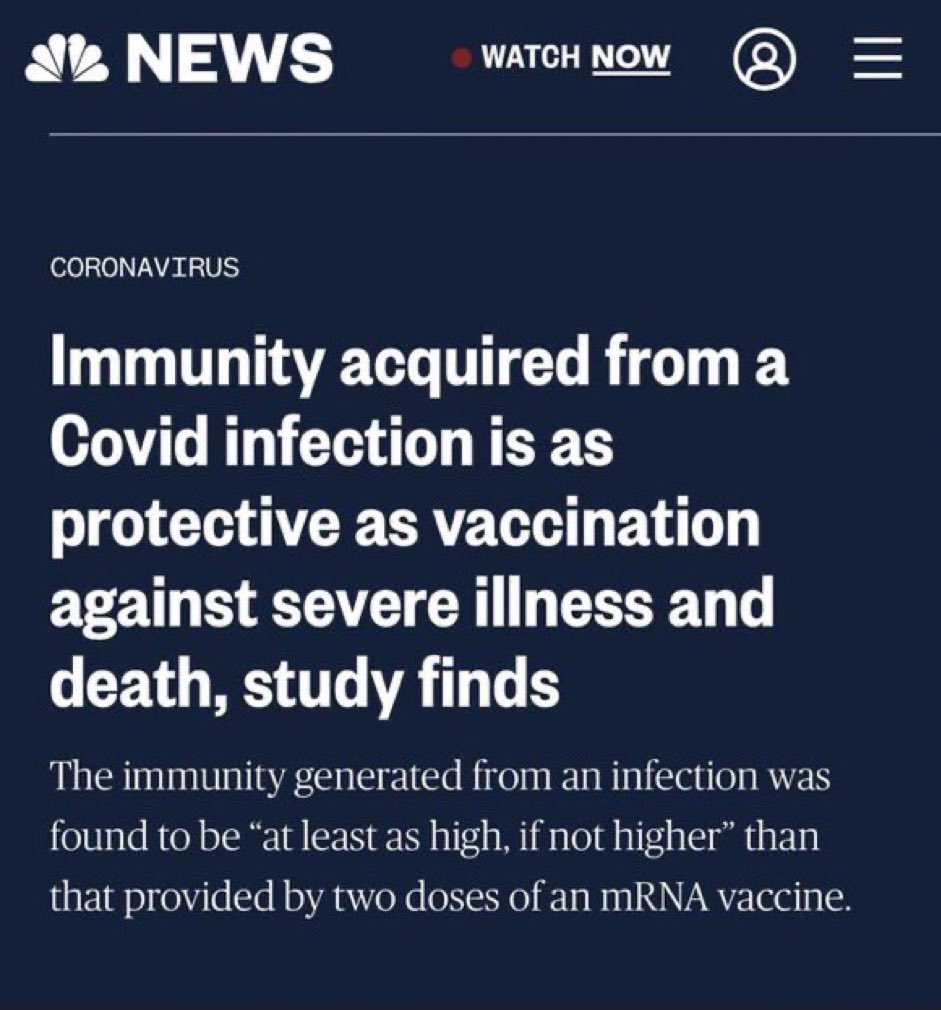In the upper left corner of the image, there is the recognizable NBC News logo, consisting of six white feather-like shapes that resemble turkey feathers. Beside the logo, in bold uppercase letters, the word "NEWS" is prominently displayed. Adjacent to "NEWS" is a red dot followed by bold text that says "Watch Now". Below this, in smaller white text, the word "Coronavirus" appears. The main headline reads in bold white text: "Immunity acquired from a COVID infection is as protective as vaccination against severe illness and death, study finds."

Below the headline, additional information is provided in lighter text: "The immunity generated from an infection was found to be at least as high, if not higher, than that provided by two doses of an mRNA vaccine," with "RNA" in uppercase letters for emphasis. At the top of the image, there is an option to "Watch Now", and a profile icon indicating the option to access a user profile if one has already been created. In the far right corner, three short horizontal lines are displayed, likely representing a menu.